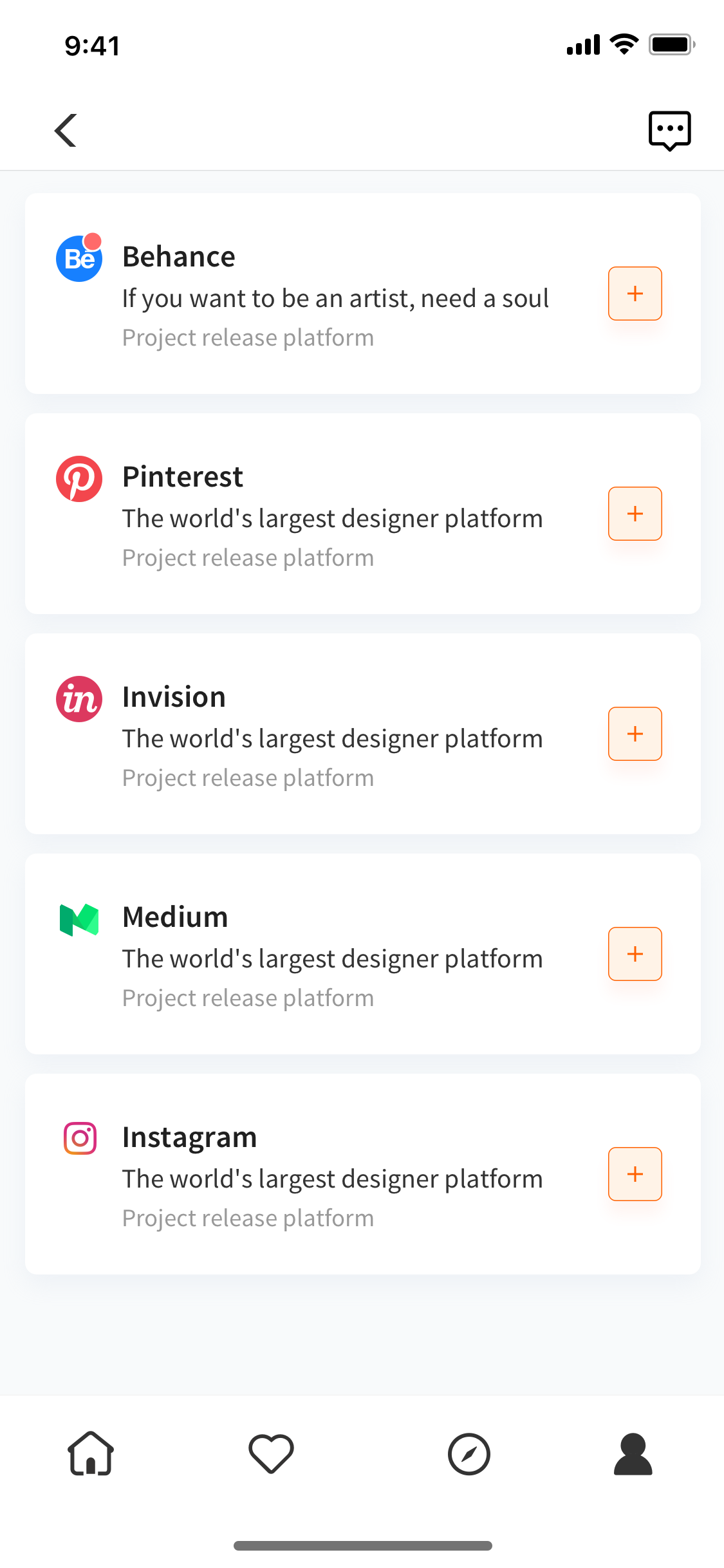This is a detailed screenshot of a mobile app interface. At the very top of the screen, the time is displayed as 9:41 on the left side, while the right side shows full signal strength and a fully charged battery. Below this status bar, there are navigational elements; a back arrow pointing left is on the left side, and a dialogue icon with three dots is situated on the right side in the same horizontal line.

Lower in the interface, there is a list of options presented in a series of rectangular boxes:

1. The first box features a blue Behance logo and reads: "Behance - If you want to be an artist, need a soul, project release platform". To the right of this box, there's a red square with a plus symbol.

2. The second box highlights Pinterest with its red logo, accompanied by the text: "Pinterest - The world's largest designer platform, project release platform". This box also has a red square with a plus symbol on its right side.

3. The third box lists Envision with a red circular logo containing the letters "IN", followed by the text: "Envision - The world's largest designer platform, project release platform". A red square with a plus symbol is positioned to the right of this box as well.

4. The fourth box showcases Medium with a green logo, alongside the phrase: "Medium - The world's largest designer platform, project release platform". A red square with a plus symbol is similarly located to the right.

5. The fifth box displays Instagram with its characteristic logo, described as: "Instagram - The world's largest designer platform, project release platform". It also features a red square with a plus symbol to the right.

Below these boxes, there is a horizontal row of four symbols: a house icon, a heart icon, a time icon, and a person icon. At the very bottom of the screen, there is a horizontal bar extending across the width of the interface.